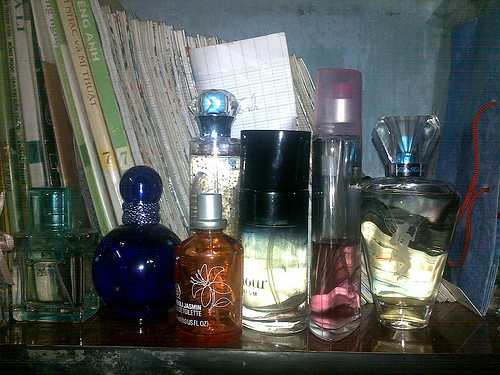On a black laminate shelf against a striped blue wall, various fancy perfume bottles are meticulously arranged, providing a sense of opulence. The shelf is cluttered, but the perfumes take prominence with their distinct and elaborate designs. 

To the far left sits a short, bluish-green fragrance bottle adorned with a nondescript picture. Next to it, a striking cobalt blue round bottle with a matching round stopper, lined with a silver rope, catches the eye. Following this is an orange bottle embellished with a lily-like flower and capped with a silver stopper. 

Further to the right, a unique glass bottle transitions from blue at the top to clear at the bottom, featuring a black stopper and subtle grayish-silver writing. Beside it, a clear bottle holds pink liquid, capped with a matching pink see-through stopper that reveals a pink atomizer. The last prominently displayed bottle is triangular with a possibly etched image of a mermaid and a blue atomizer inside, its topper mimicking the triangular shape in a corrugated style.

Interspersed with these perfumes are several books and magazines, some having visible spines numbered 7 in off-white and green colors. The overall scene exudes a sense of luxury and sophistication, despite the poor lighting and the somewhat chaotic arrangement.